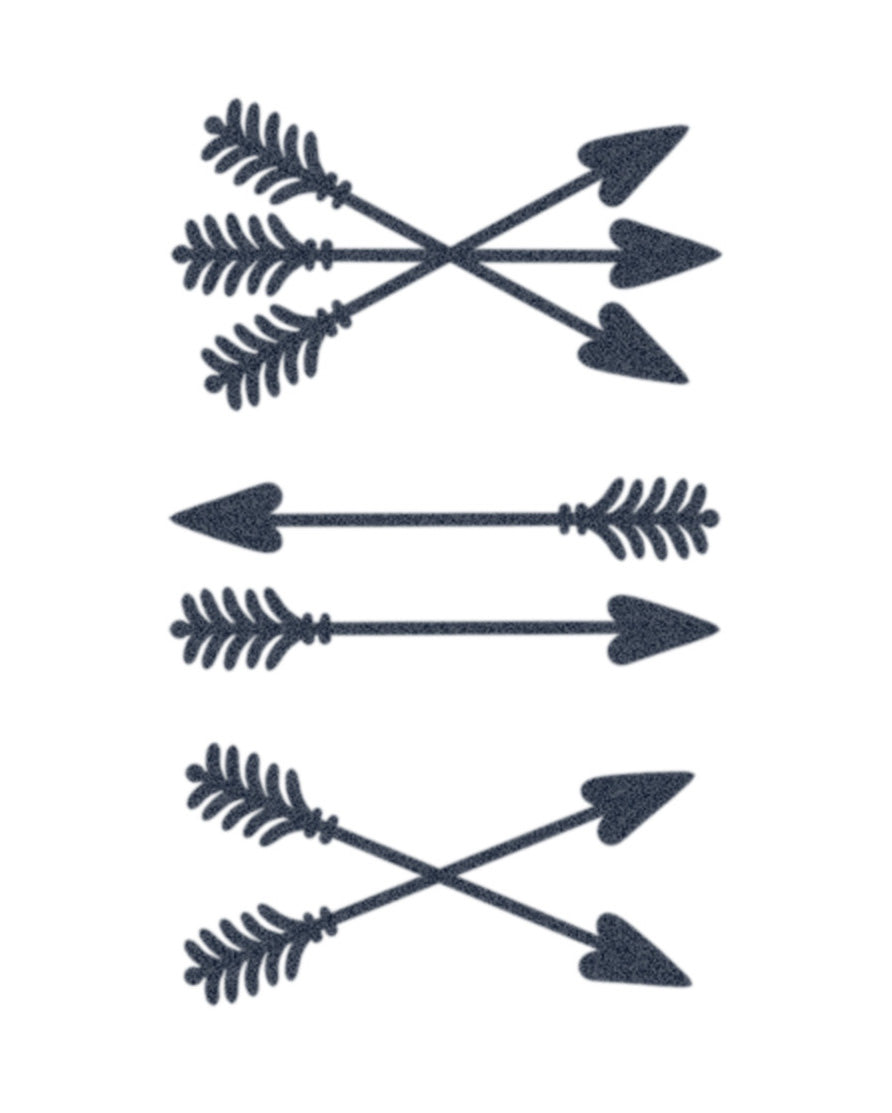The image is a detailed illustration featuring a series of intricately designed arrows, set against a plain, empty background. Each arrow has a distinctive heart-shaped end and is colored in a mottled black and blue, giving them a metallic appearance rather than the traditional feathered look.

At the top of the image, there are three large arrows overlapping in the center, each pointing in a different direction: one upwards, one horizontally to the right, and one downwards. Below this top arrangement, the middle section depicts two arrows positioned horizontally and pointing in opposite directions - one to the right and one to the left. Finally, at the bottom of the image, there are two arrows that intersect in an X shape, with their tips pointing towards the right.

The composition of the arrows – their intricate details and metallic finish – along with the absence of any background context, draws full attention to their arrangement and forms.